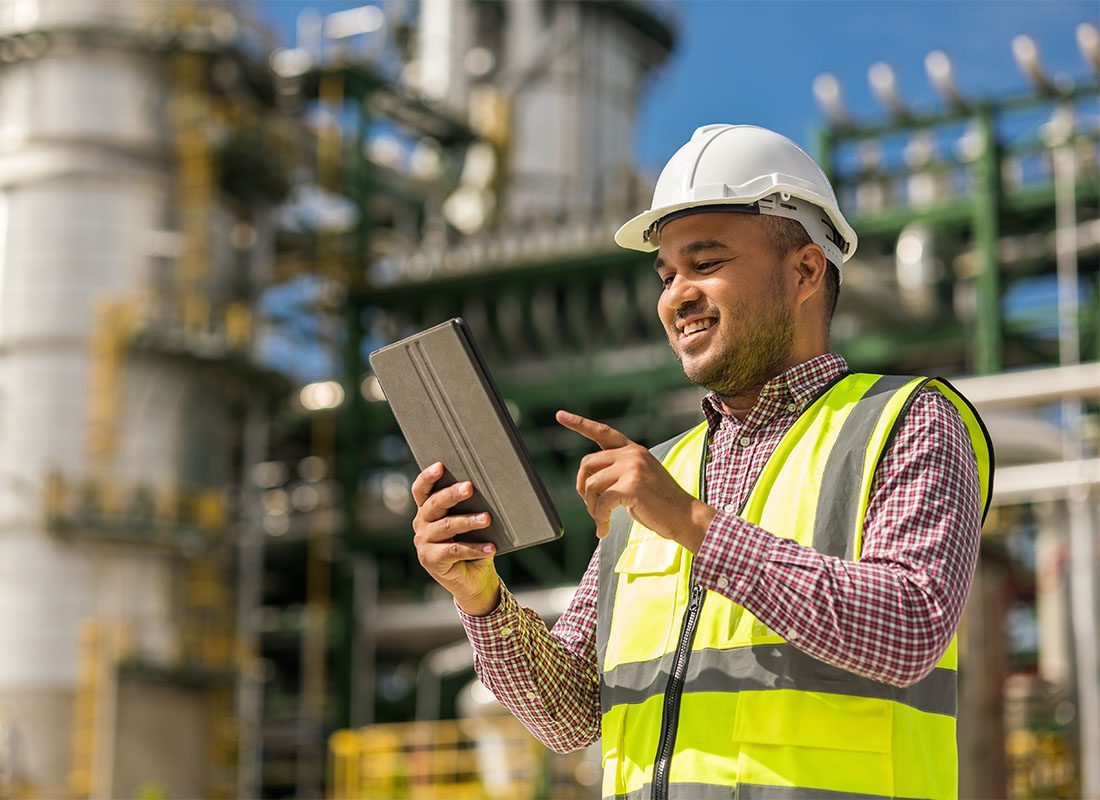In this bright and detailed photograph, a construction worker, who appears to be of either Latino or Arabic descent, stands confidently at a job site, likely a power plant or a similar industrial facility. He is captured smiling as he holds a tablet, possibly an iPad, in his right hand while his left index finger hovers close to the screen, suggesting he's about to interact with it. He is dressed in a vibrant yellow safety vest over a red and white plaid long-sleeved shirt, and his head is protected by a white hard hat. Behind him, a large cylindrical structure, possibly a silo or vat, is blurred, adding context to his surroundings without detracting attention from his focused expression and engaged demeanor. His tan or dark olive-toned skin complements his close-shaved beard, further emphasizing his professional and approachable appearance.